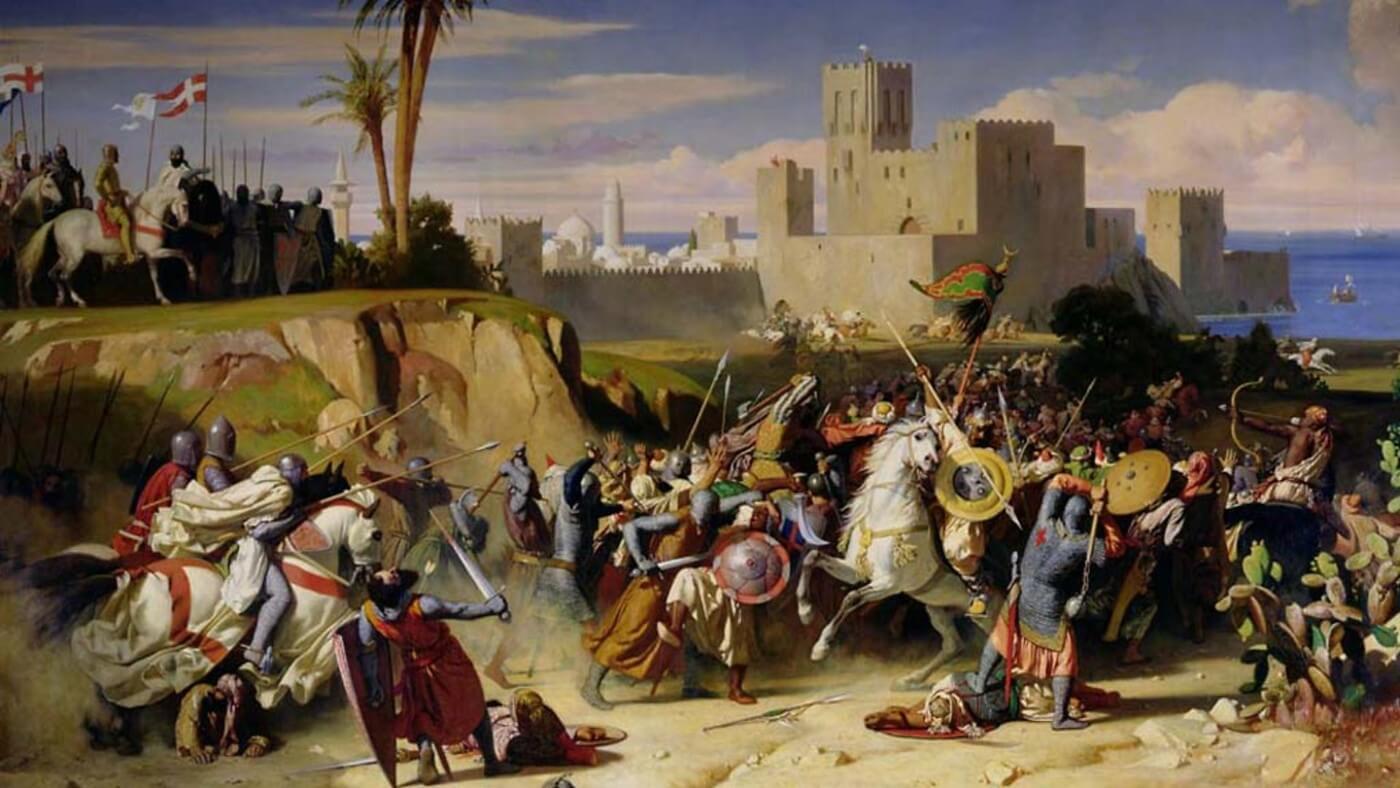The painting depicts a chaotic, vividly detailed battle scene likely featuring conquistadors. Dominating the foreground, numerous soldiers—both on horseback and on foot—clash intensely with a myriad of weapons, including spears, bows and arrows, knives, and axes. The heavily armored knights, distinguishable by their ornate heraldry of white crosses on a red field and red crosses on a white field, ride horses draped in colorful cloth. On the right, darker-complexioned archers also join the fray, with cactus plants visible nearby. The left side of the composition features a small hill or plateau with additional soldiers observing the turmoil below, signaling tactical movements. In the background, a majestic walled city extends partially into the sea, with domed buildings and a castle silhouetted against the sky and clouds. Palm trees scatter the landscape, adding to the exotic atmosphere, while a small boat sails on the water, further enriching this dynamic portrayal of historical warfare.